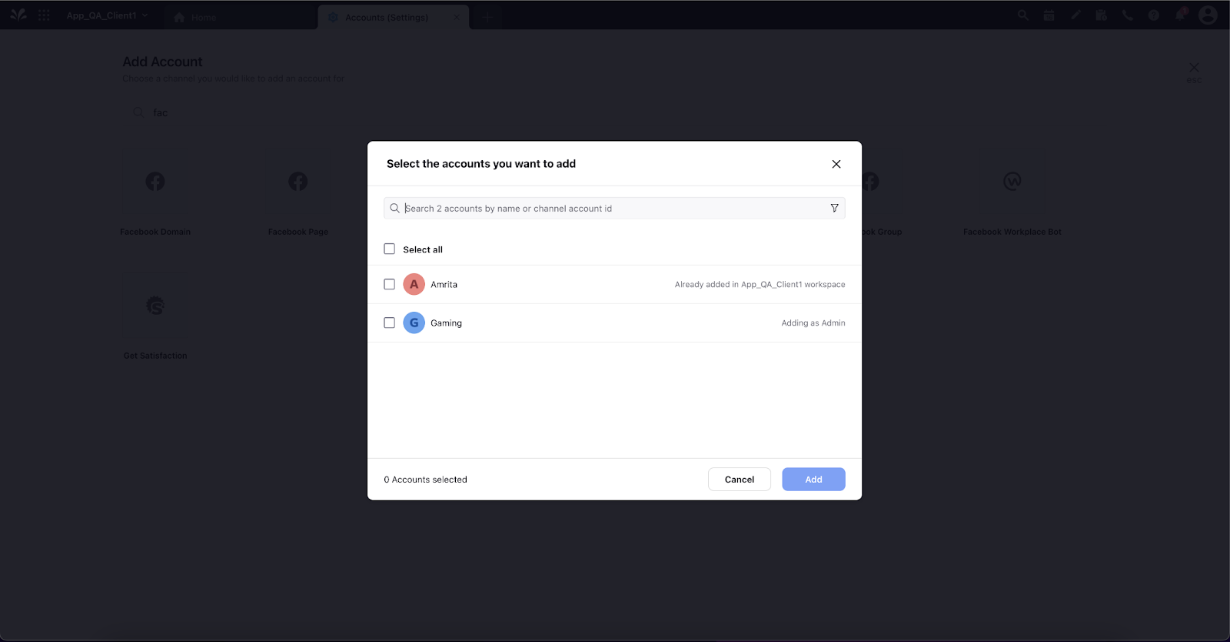The image depicts a screenshot of a computer screen, specifically showing a pop-up window at the center. This window is titled "Select the accounts you want to add," with an 'X' button on the far right to close the pop-up. At the very top of this window is a search bar labeled "Search accounts by name or channel, account ID," with a small tornado icon at its endpoint.

Below the search bar is a checkbox labeled "Select All." Two accounts are listed beneath this option: one annotated with an 'A' for "Amvita" and another with a 'G' for "Gaming." Both accounts have checkboxes next to them for selection. The account labeled 'A' includes a note indicating it is "Already added in app_QA_client1 workspace," while the account labeled 'G' has a note reading "Adding as admin."

Towards the bottom of the window, a message states "0 accounts selected," indicating no accounts have been chosen for this action. Finally, two buttons are visible at the bottom of the pop-up window: one labeled "Cancel" and the other labeled "Add."